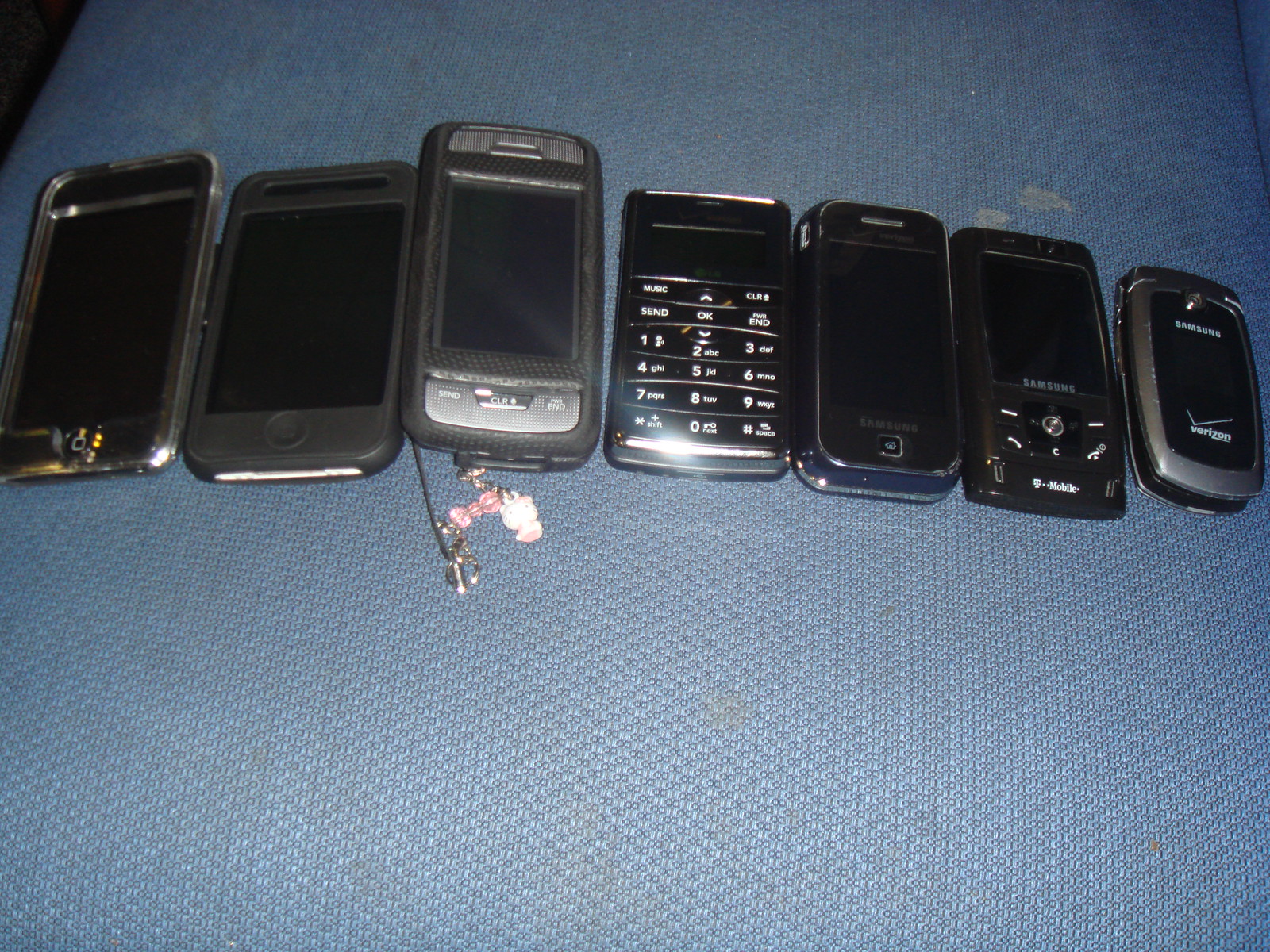The image depicts a collection of seven old cell phones carefully lined up from left to right on a worn, blue cushion of a couch. The lineup begins with a gray flip phone, followed by a black BlackBerry, then a blue flip phone, and another black device resembling a newer BlackBerry. The arrangement transitions into early smartphones, including at least two iPhones—one in a clear case and the other in a silicone case. Among these, there are three Samsung phones, alongside individual models from LG, Verizon, and T-Mobile. The couch cushion they rest upon is notably dirty, marred with various stains, including prominent white stains above the phones and brown stains below. Particularly distinctive is the third phone from the left, which is pink and adorned with a decorative chain or charm bracelet.